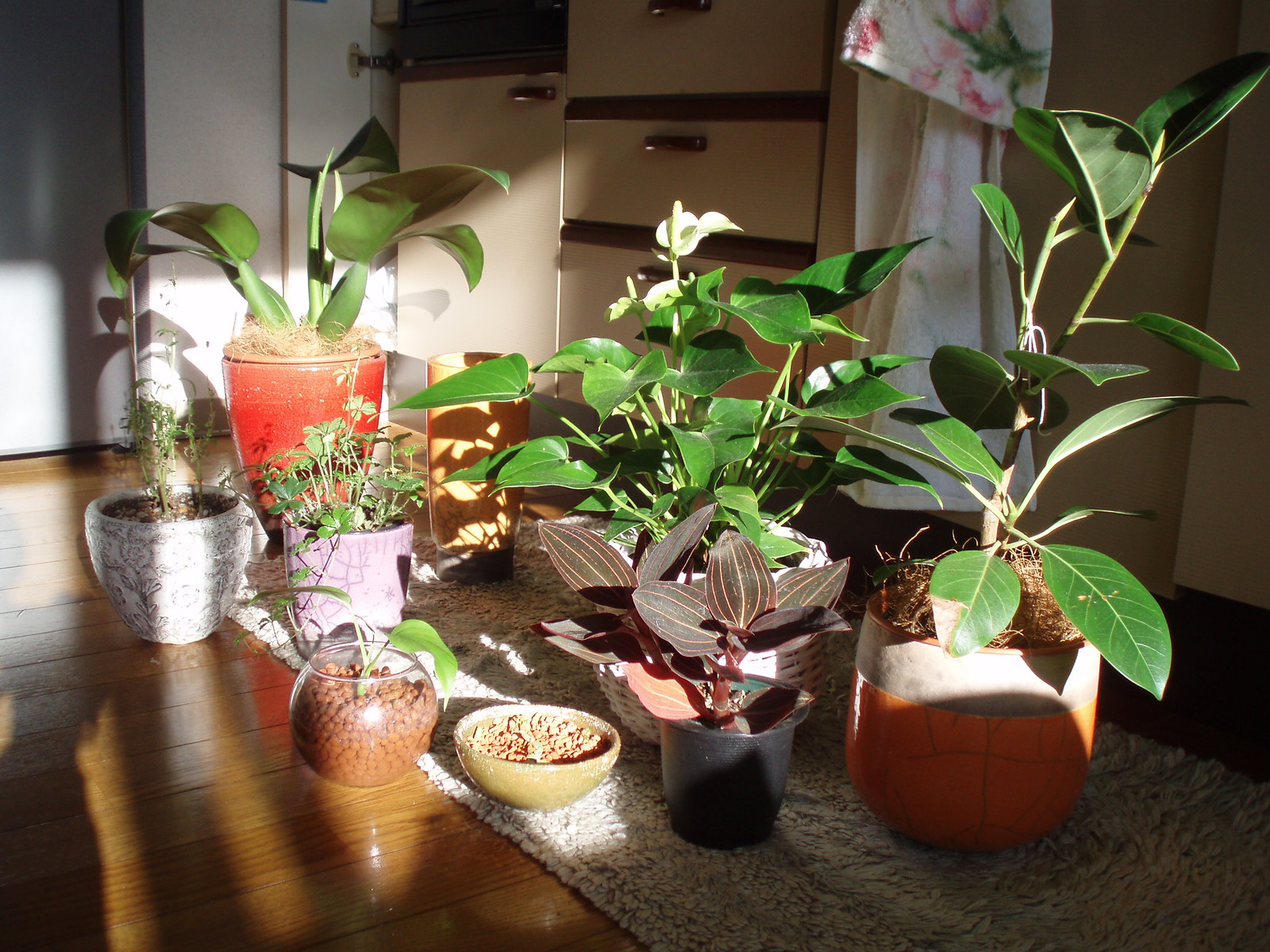This colored photograph captures an indoor scene bathed in vibrant, splotchy sunlight, likely filtering through a window or an open door. The setting suggests it's a kitchen, evident from the blurry kitchen cabinets and a doorway visible in the background. The sunlight casts dramatic patterns on a grouping of around ten potted plants, some placed on a rug and a couple on the wooden floor. The pots themselves vary in colors and materials—including pink, light gray, brown, black, blue or purple, orange, red, and even glass. 

The plants exhibit diverse types and sizes, with broad green leaves dominating the scene. There are a few distinctive plants, such as one resembling a lily and another akin to elephant ears, while some feature darker reddish-black leaves with red lines. Despite the variety in leaf colors—ranging from green to shades of brown and red—no flowers are visible on the plants. This assortment, potentially set out for watering or sunlight exposure, contributes to a lively and eclectic indoor garden ambiance.